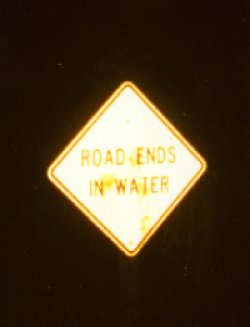The image captures a prominent yellow, diamond-shaped sign with a bold black text stating "ROAD ENDS IN WATER." This reflective warning sign, likely illuminated by headlights or another bright light source, stands out against a pitch-black background, suggesting it was taken at night. The sign features a brighter, highly reflective yellow interior with a deeper orange or yellow border that is less reflective. Notably, the sign shows signs of wear, with yellow and brown stains, indicating its age. The photograph itself appears vintage, marked by a grainy, old-fashioned quality with a yellowish tint. The sign is mounted on a pole, although the pole and surrounding environment remain obscured by darkness. The illuminated reflection and the smudges present on the sign, particularly between the words "IN" and "WATER," add further detail to its weathered appearance.